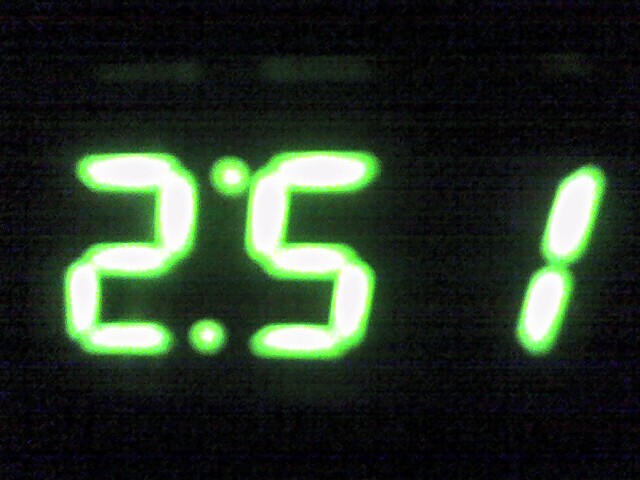The image features a black background with faint, indistinguishable print or pattern spread across the center from left to right. Dominating the image are a series of numbers in the middle left area, each depicted in bright white and outlined in neon green, giving them a glowing effect. Starting from the top left, there is a number '2', followed by two small dots situated nearby. Next, there is a number '5', also in white with a neon green outline. After a noticeable gap, a number '1' appears with the same color and outline effect. The barely visible background print adds a layer of mystery, hinting at hidden elements behind the brightly illuminated numbers.